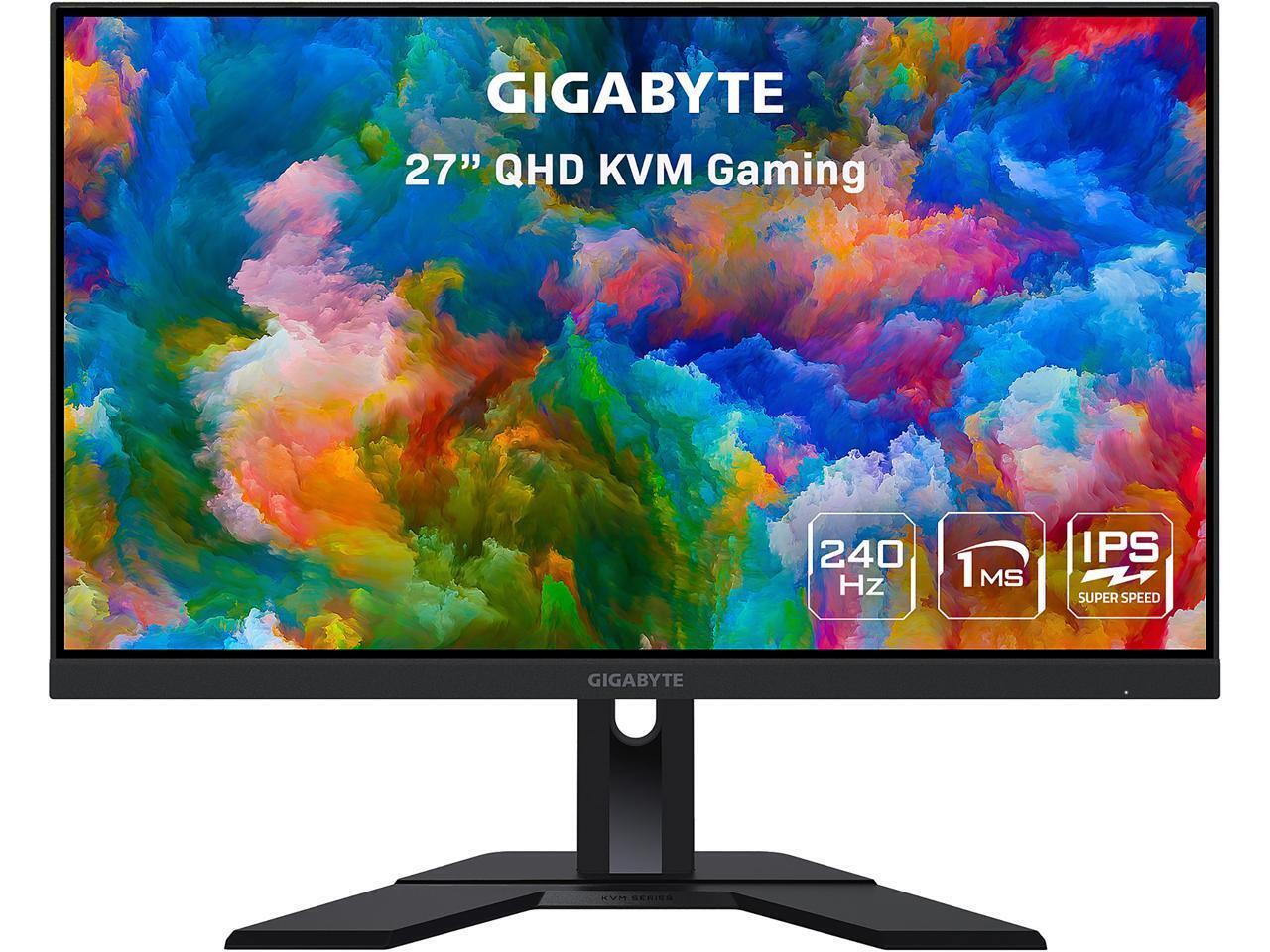This image depicts a black-framed Gigabyte computer monitor with a black plastic base situated on a white background. The screen prominently displays the word "Gigabyte" at the center in gray text, along with the specifications "27 inches QHD KVM gaming." In the bottom right of the screen, there are four white logos arranged in squares, detailing the monitor's key features: "240 Hz," "1ms," "IPS," and "Super Speed" with an accompanying lightning bolt arrow. The screen shows a vibrant, multicolored cloud-like or marbled pattern using hues of blue, green, orange, pink, purple, and red. The top of the monitor touches the top edge of the image, with indistinct borders on the sides and bottom, adding to the modern and colorful presentation of the monitor's capabilities.